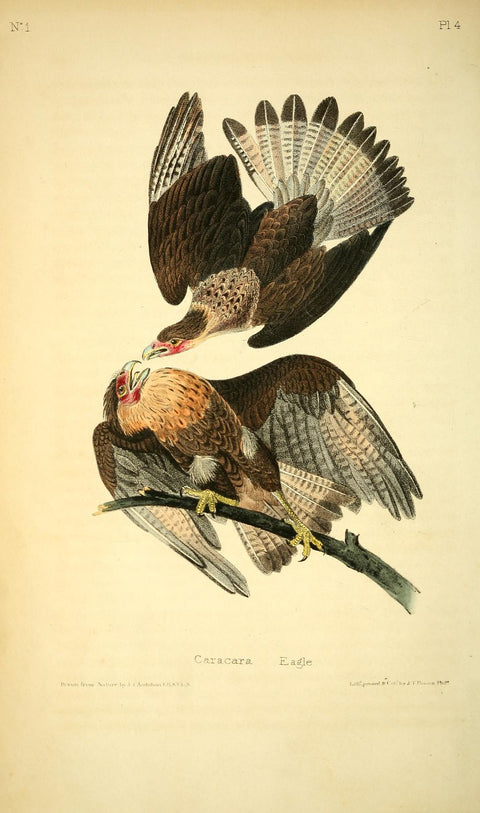This vintage art print, set against a worn, beige paper backdrop, depicts a detailed scene of two brown Caracara eagles in a dynamic interaction. The top left corner is marked with "N1," and the top right with "PL4," while below the image, in faded gray text, it reads "Caracara eagle." The illustration, which appears hand-drawn with colored pencils or possibly painted, shows two birds with large beaks and claws. Both have red faces and white-speckled feathers. The eagle perched on a black branch has its wings spread, displaying yellow legs, an orange belly, and striped gray and white wingtips. Its posture suggests it's preparing to defend against the second eagle, which is swooping down with its beak open, seemingly about to make contact. The swooping eagle mirrors the perched one's coloration, with brown wings, a red face, and white tail feathers tipped in black. This print, resembling something one might find in a history book or museum, vividly captures the fierce encounter between the two majestic birds.